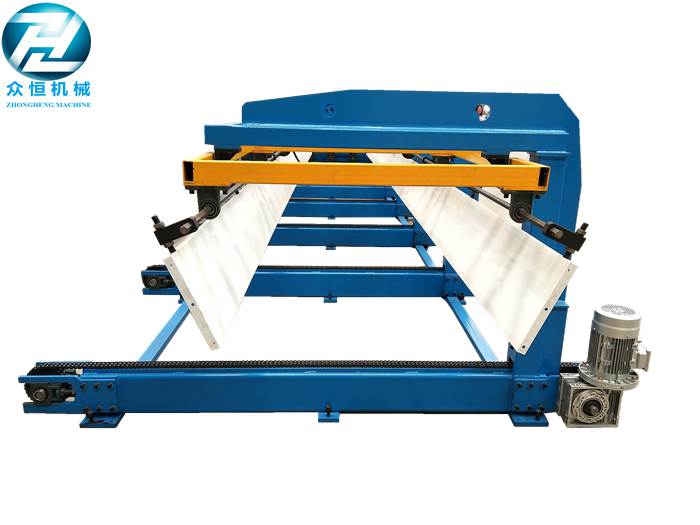The image showcases an intricate piece of industrial equipment set against a stark white background, which makes the vibrant blue machinery stand out prominently. In the upper left corner, there is a blue and white interlocking logo featuring the letters ZH and some non-English characters, along with the name "Zongchang Machine" inscribed below. The main apparatus resembles a complex tow dolly or pulley mechanism, incorporating several bays or sections that extend into the distance. The structure is primarily composed of metallic blue beams and includes yellow bars that descend from an overhead arm. Additionally, there are white rollers or runners hanging down from the sides, while a silver engine or compressor-like component is situated at the bottom right of the machinery. The overall layout suggests a highly specialized machine, rich in metallic textures and intricate operational parts.